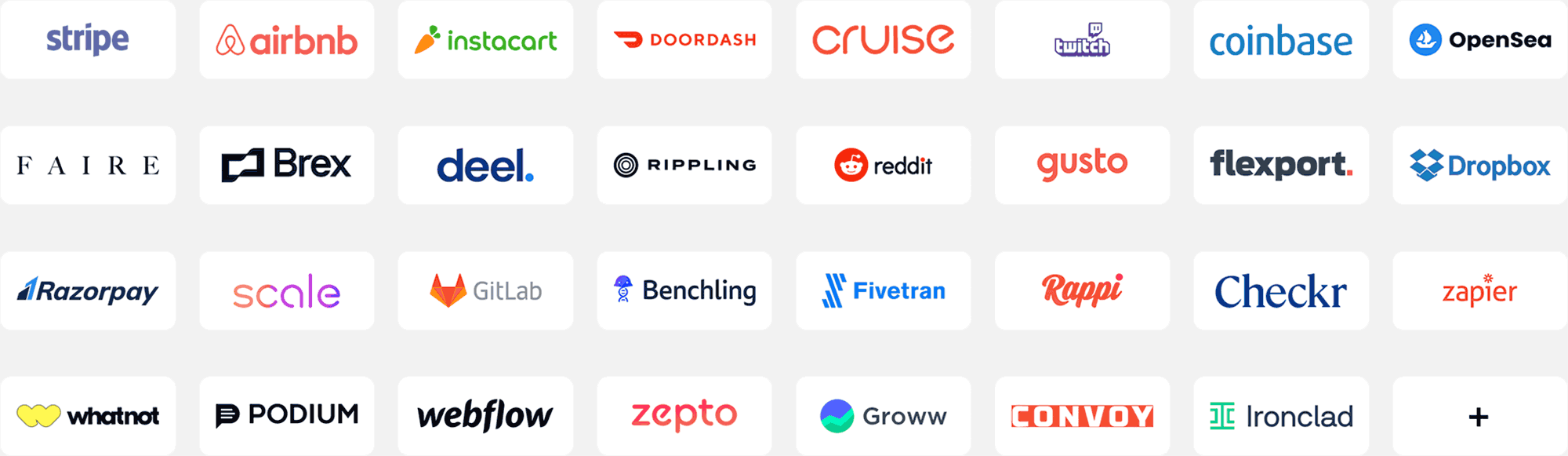The image showcases a neatly arranged grid of various business logos, each encased in white rectangular boxes. The logos are organized into four rows, with each row containing up to eight logos. The first row features Stripe, Airbnb, Instacart, DoorDash, Cruise, Twitch, Coinbase, and OpenSea. In the second row, the businesses displayed are Faire, Brex, Deel, Rippling, Reddit, Gusto, Flexport, and Dropbox. The third row includes Razorpay, Scale, GitLab, Benchling, Fivetran, Rappi, Checkr, and Zapier. The final row consists of Whatnot, Podium, Webflow, Zepto, Grow, Convoy, and Ironclad, with the last box featuring a plus sign, suggesting the possibility to add another logo. Each business logo is presented with distinct colors, such as Coinbase in blue and Cruise in red, set against a light gray background, highlighting their unique identities.